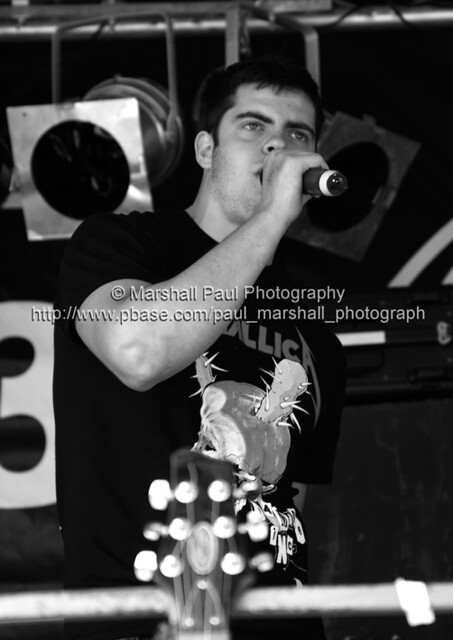In this striking black and white photograph taken by Marshall Paul Photography, a young male singer with short dark hair intensely performs in a concert hall. Captured with a serious expression, he holds a microphone close to his mouth with his left arm slightly raised. He wears a black t-shirt featuring a design and the letters "C-L-I-C," which might have slightly blended with the watermark text. 

In the foreground, the blurred guitar headstock, complete with tuning pegs, rests against a cylindrical metal railing at the singer's waist level, hinting at the musical ambiance. The background remains dark, adding to the dramatic focus on the singer, while two inactive spotlights hover behind him, suggesting a professional concert setting. A watermark imprinted across the center reads "Marshall Paul Photography, http://www.pbase.com/paul_marshall_photograph," crediting the photographer's work.